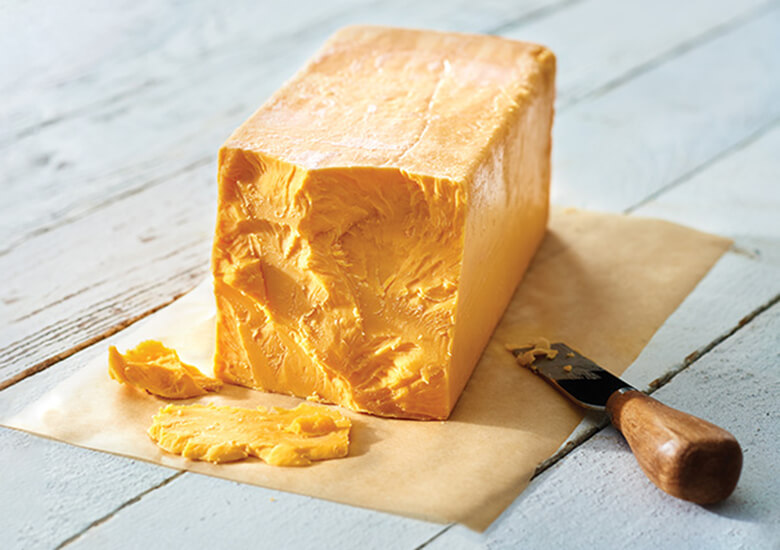The image features a large, rectangular block of orange-yellow cheese, likely cheddar, displayed on a piece of brown parchment paper. This setup rests on a weathered white wooden surface, which appears to be either a table or wooden slats. The front of the cheese block has several cuts, including two prominent, uneven chunks that seem to have been roughly torn off, suggesting a less precise method of removal. A cheese knife, characterized by its dark metal blade and brown wooden handle, lies flat in the lower right-hand corner of the composition. The blade bears remnants of cheese, indicating its recent use. The background of the image is blurred, drawing focus to the detailed textures and colors of the cheese and cutting implements.